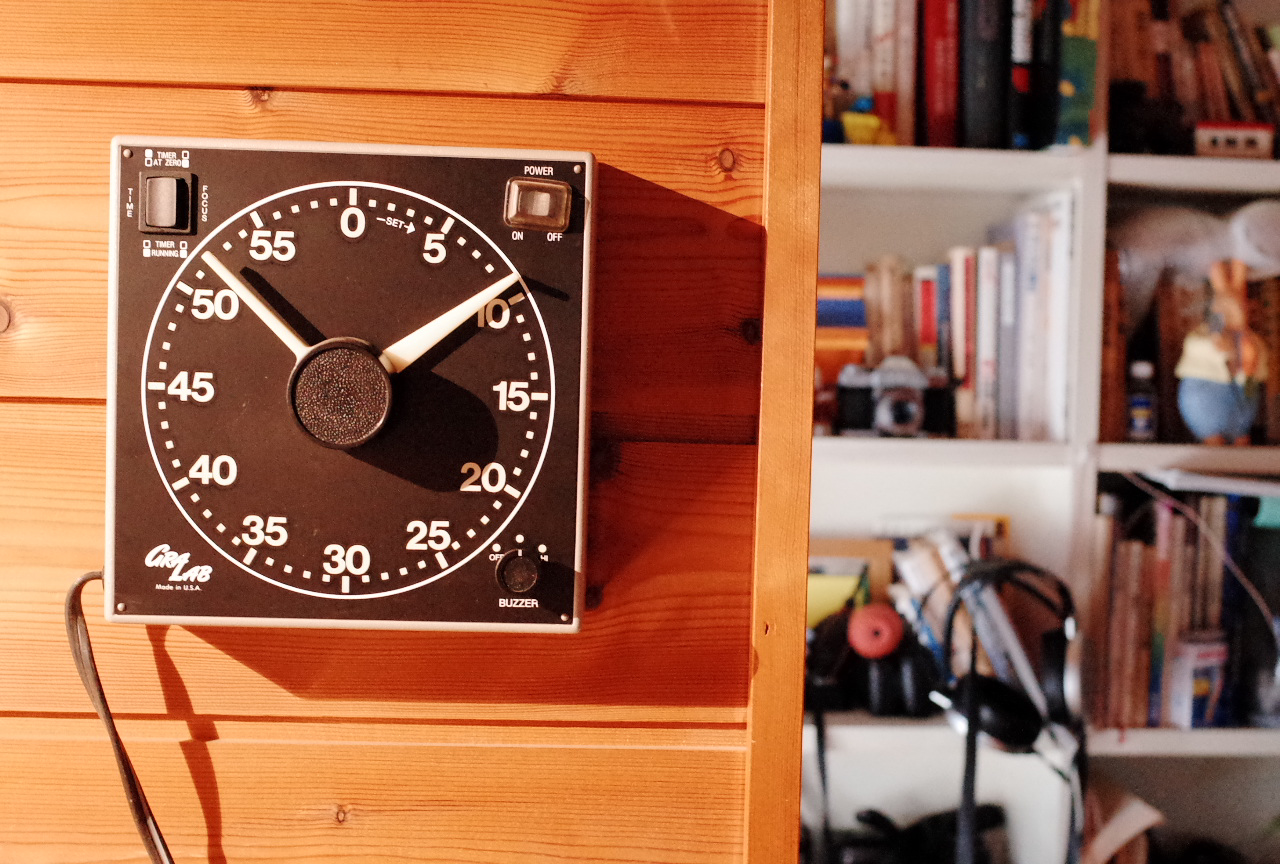A detailed caption of the image:

On the left side of the image, there is a rusty brown wall, partially showcasing the texture of the wood. Mounted on this wall is a black instrument that resembles a compass, featuring numbers marked in increments: 0, 5, 10, 15, 20, 25, 30, 40, 45, and 50, with white numbering. The center button of this device is brown, and it has white hands, which are currently pointing to 52 on the left side and 9 on the right side. 

At the top left corner of the device, there is a button with indecipherable words. On the top right side, a power button is clearly labeled "POWER," with "ON" noted on the left bottom part of the power button and "OFF" on the right bottom part. Below the power button, at the lower left-hand corner, there is a label that reads "MADE IN USA," though the name above it is not legible. 

On the lower right-hand side of the device, another button reads "BUZZER" beneath it. This button is outlined in white and features three additional settings marked by dots. A wire protrudes from the lower left-hand side of the device, but it is cut off in the picture.

The right side of the image appears to be a closet or storage area with shelving. These shelves are filled with various items, including books, toys, and a camera among other miscellaneous objects.